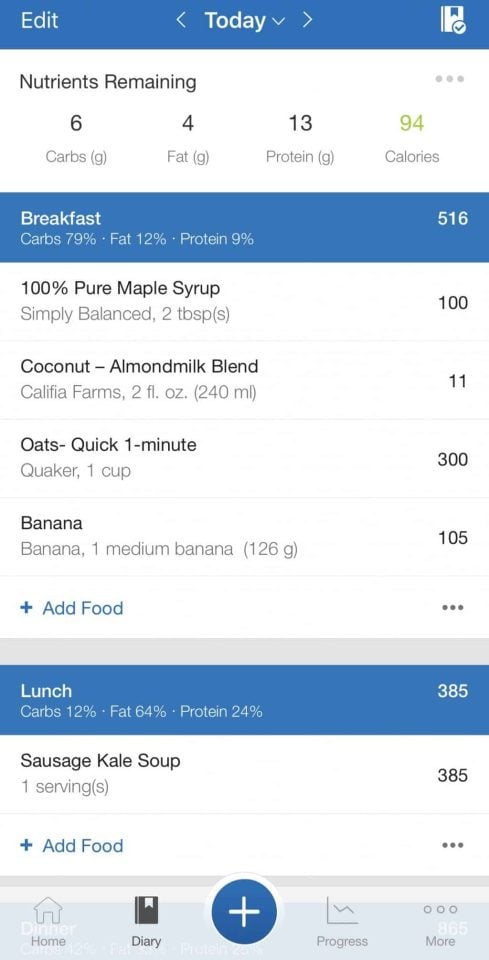The image showcases a calorie-tracking app with a white background. At the top, the header features a blue background with white text that reads "Edit" in the top left corner and "Today" centered. Below this, the app displays "Nutrients remaining: 6g carbs, 4g fat, 13g protein, 94 calories," with the calorie count highlighted in green while the other numbers are in black.

Beneath, the section labeled "Breakfast" shows a total of 516 calories, broken down into 17% fat, 12% protein, and 9% carbs. Below this, there's a detailed list of breakfast items:

- 100% Pure Maple Syrup, Simple Balanced, 2 tablespoons: 100 calories
- Coconut Almond Milk Blend, Cauliflower Farms, 2 oz (240 ml): 11 calories
- Quick 1-Minute Oats, Quaker, 1 cup: 300 calories
- Banana, 1 medium (126 grams): 105 calories

A blue "Add Food" button is located beneath the breakfast section.

Further down, the "Lunch" section totals 385 calories with macronutrients detailed as 12% carbs, 64% fat, and 24% protein. The listing includes:

- Sausage Kale Soup, 1 serving: 85 calories

Another blue "Add Food" button is positioned below the lunch information.

At the bottom of the app, a navigation bar features buttons for Home, Diary, Add (center, blue), Progress, and More.